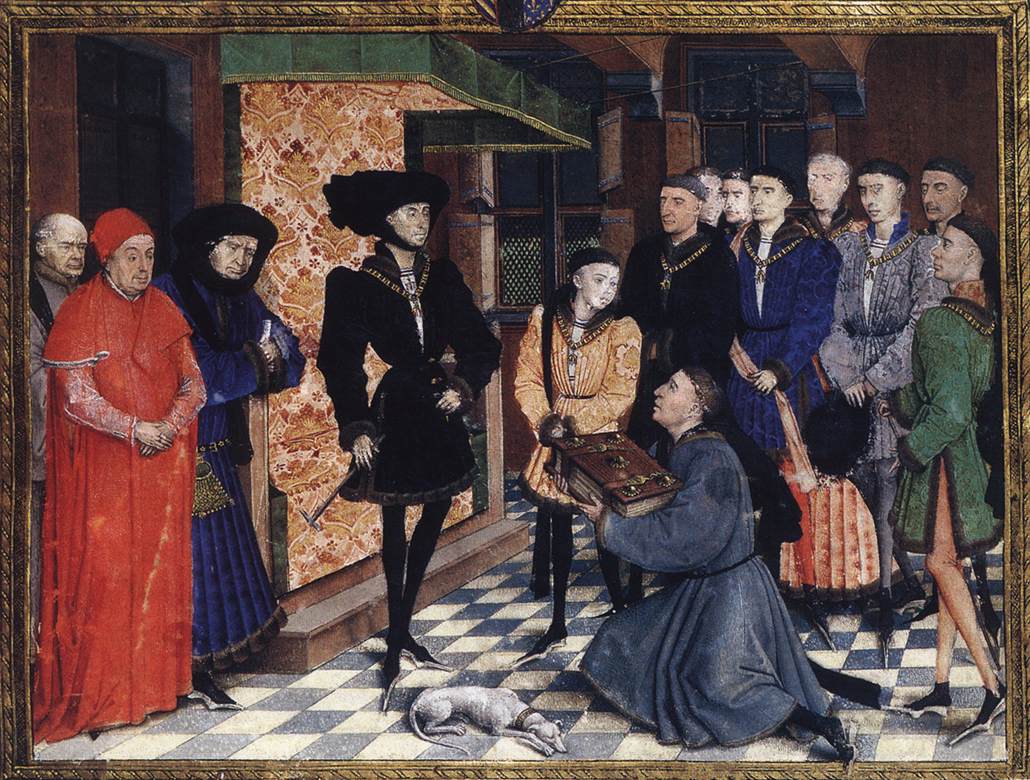In a goldish-brown frame, this painting depicts an elaborate indoor scene with a checkered blue and white tiled floor. At the center, a man draped in a black outfit, adorned with an ornate hat and jacket, holds a significant presence. He is gazing slightly to the right and forward. Directly in front of him, a monk-like figure with short black hair kneels, holding a thick, strap-bound, brown book, revealing its white pages. The monk, wearing a gray robe and a skull cap, is observed by several onlookers.

To the monk's left, three figures stand: one in a flowing red robe and matching cap, with hands folded in front; another in a black and blue cape; and a bald man, partially obscured, behind them. To the monk's right lies a white dog, adding a touch of domesticity to the ceremonious setting. Near this central figure, stands a shorter person in a black cap and beige outfit with poofy sleeves, facing the monk.

Further right, a group of eight or nine individuals in various attire—ranging from black, blue, green, to gray-colored robes—look towards the kneeling man. The background showcases a tapestry-like wallpaper in beige with dark accents, contributing to the sense of grandeur. The detailed attire of some figures, featuring necklaces and skull caps, hints at a ceremonial gathering, potentially in the interior of a church or a castle.